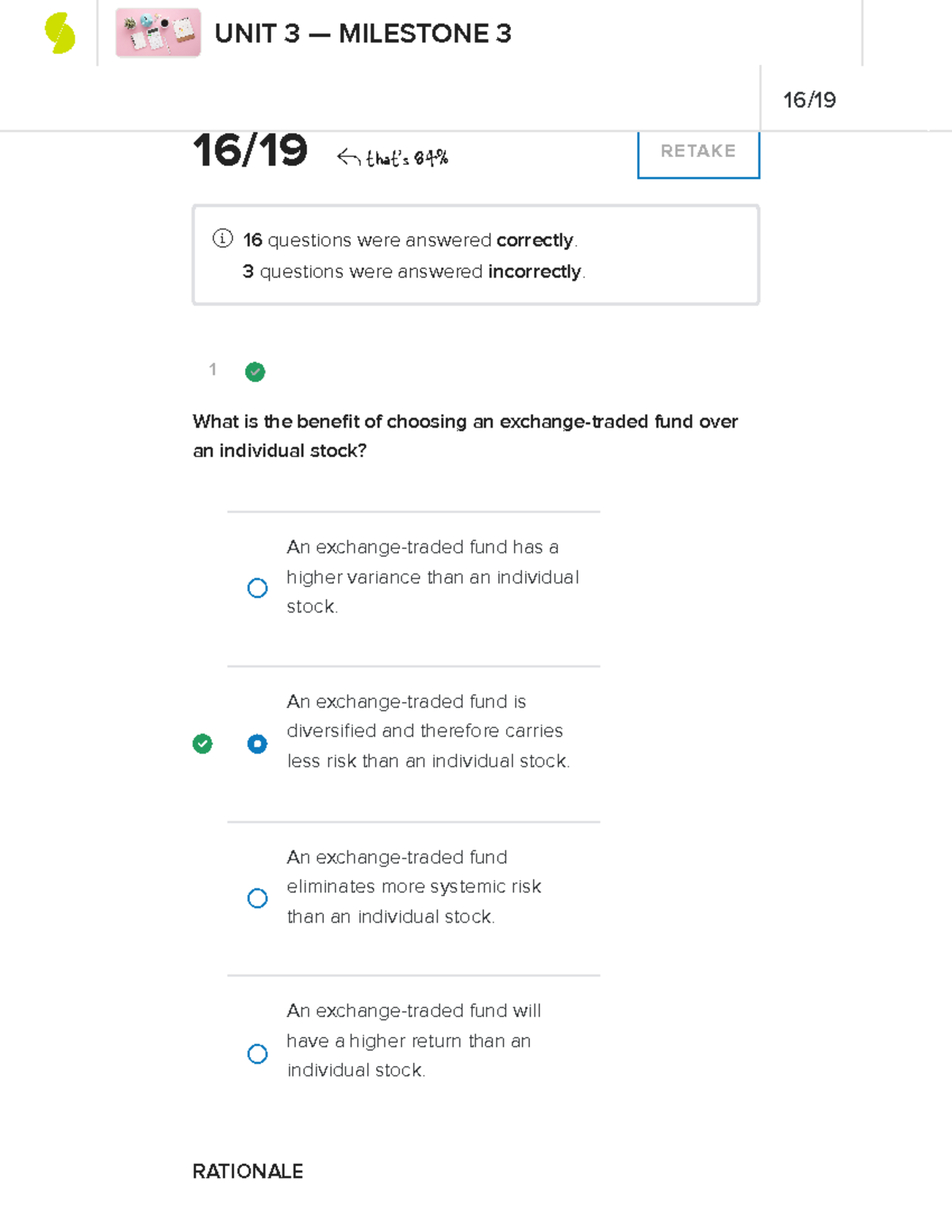The image displays a user interface from an educational or assessment platform. At the top, there is a stylized graphic resembling a split circle with lines that create an "S" shape due to the segments being offset from each other. Adjacent to this graphic are what appear to be representations of writing tablets, which could signify saved work or milestones achieved.

To the right of these graphics, the following text is displayed: "Unit 3 - Milestone 3" followed by "16 of 19," which likely indicates the user's progress through the milestone (16 questions answered out of 19 total). Adjacent to this is a progress indicator expressed as "84%," accompanied by a backward-facing arrow.

The current tab displayed is titled "Retake," suggesting the user is reviewing or retrying their answers. Below this tab, within a faint gray box featuring an information icon, text indicates that "16 questions were answered correctly" and "3 questions were answered incorrectly."

Further down, a list of questions and their corresponding answers is shown. The first displayed question is, "What is the benefit of choosing an exchange-traded fund over an individual stock?" Below this question, several faint gray lines separate multiple-choice options:

1. "An exchange-traded fund has higher variance than an individual stock." (This option is unselected and marked with a bubble).
2. "An exchange-traded fund is diversified and therefore carries less risk than an individual stock." (This option is selected, indicated by a green circle with a white check and a blue bubble that is checked).
3. "An exchange-traded fund eliminates more systemic risk than an individual stock." (This option is unselected and marked with a bubble).
4. "An exchange-traded fund will have a higher return than an individual stock." (This option is unselected and marked with a bubble).

At the very bottom, the section labeled "Rationale" likely contains explanations or justifications for the correct answers.